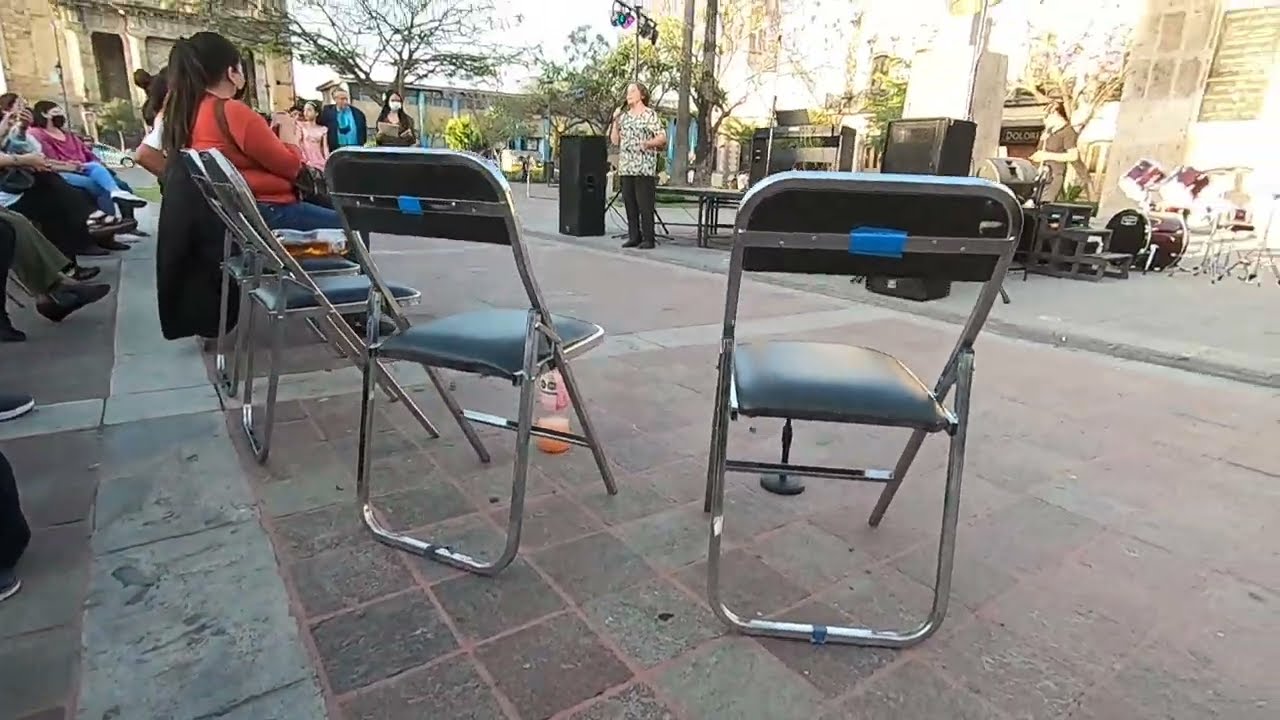In this outdoor scene captured in a horizontally aligned rectangular photograph, a group of people are seated on teal blue folding chairs with metal legs that form a semicircle around a female speaker. The sidewalk, composed of brown and gray square bricks, hosts this gathering on a bright and sunny day. The speaker, dressed in a patterned white and black top, black pants, and black shoes, holds a microphone and stands before a set of large black speakers and a drum set. Behind her, lights and additional sound equipment are visible, poised for potential use during what appears to be a preparatory stage for a musical performance.

Among the audience, seated in neat rows, is a woman with long dark hair tied back in a ponytail, donning a red shirt. Another attendee, discernible by her dark hair and face mask, sits observing the speaker. Off in the upper left of the image, a woman with long brown hair gathered in a ponytail and wearing an orange shirt paired with jeans is seated and also directing her attention towards the speaker. 

Behind the stage area, a cityscape of buildings can be seen along with a few green trees in front of them, adding to the picturesque environment. The scene suggests an anticipation for an event, with all eyes fixed on the speaker who addresses the audience from the center of this lively, outdoor setting.